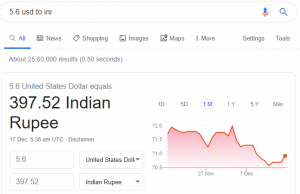A small image displayed on the screen measures approximately two inches wide by an inch and a half high. At the top of the image is a search bar, where the text "5.6 USD to INR" has been entered. Adjacent to the search bar, on its right side, are icons of a microphone and a magnifying glass, indicating voice search and the standard search option respectively.

Below the search bar, there is a multicolored magnifying glass icon, followed by the word "All" in blue with an underline beneath it. To the right, the menu options include "News," "Shopping," "Images," "Maps," "More," "Settings," and "Tools," each accompanied by their respective icons.

Further down, it displays "About 2,560,000 results (0.50 seconds)" indicating the total number of search results and the time taken to generate them. The primary result box showcases the conversion, stating "5.6 USD equals 397.52 INR" with the figure "397.52 INR" prominently in larger black font. Beneath this conversion, in smaller font, it mentions "17 Dec, 5:36 AM UTC" along with a disclaimer.

To the right of the conversion result, a graph illustrates the currency fluctuation over a period of time. The x-axis includes dates such as "27 November" and "7 December," while the y-axis marks values "70.5," "71," "71.5," and "72." The red graph line trends downward from left to right. Above the graph, there are time frame options: "1D," "5D," "1M," "1Y," "5Y," and "Max." 

This detailed layout provides a comprehensive view of the currency conversion and the historical trend of the exchange rate.